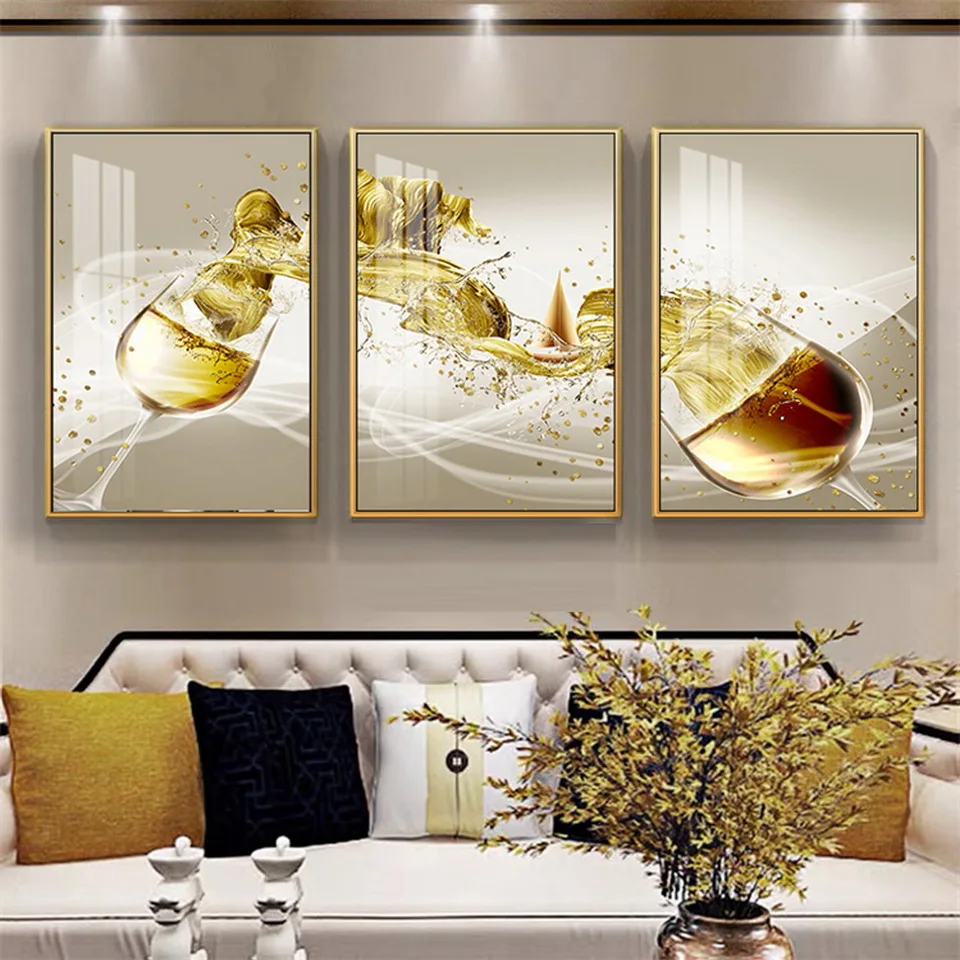The image depicts a sophisticated and possibly digitally generated living room or lounge area, characterized by a minimalist yet elegant design. Dominating the composition is a series of three gold-rimmed artistic frames mounted on a grey wall. Each frame features a photograph of a wine glass in various stages of pouring and spilling wine that flows dynamically from one image to the next, creating a sense of motion and continuity across the trio. Below these frames is a pristine white couch adorned with five pillows—two golden, two black, and one central white cushion. To the right of the couch rests a vase filled with golden flowers, lending a touch of color and natural texture. On the left, two white ceramic pieces, resembling candle holders or possibly salt and pepper shakers, complete the tranquil yet luxurious setting.